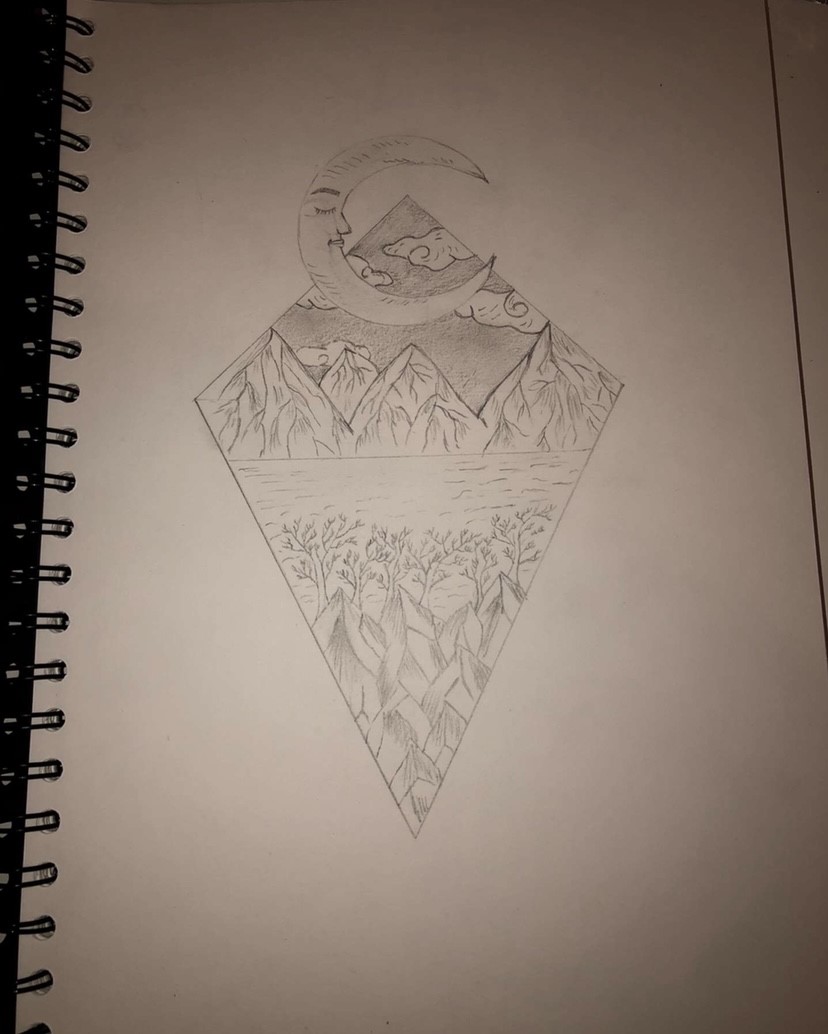In this photograph, we see an intricate pencil drawing within a spiral-bound sketchbook. The artwork is centered around a diamond shape that encapsulates a richly detailed scene. At the top side of the diamond, mountains rise majestically, topped by a serene sky. Just below the mountains, a tranquil body of water stretches across the middle of the diamond. Descending further, additional mountains appear, these adorned with small, delicate trees. At the very top of the diamond, a captivating moon with a face—complete with a closed eye, nose, and mouth—seems to be in a peaceful slumber. The image contains no text, allowing the artistry to speak entirely through its meticulous details and composition.